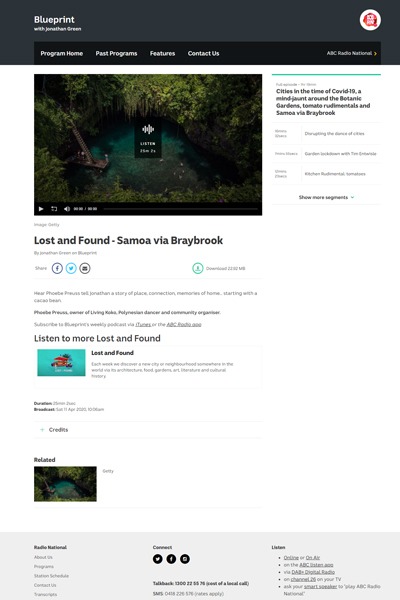Here's a cleaned-up and detailed caption for the image described:

---

The web page displayed has a dark-themed background at the top, with white text in the top-left corner reading "Blueprint with Jonathan Green." Directly below this title are several navigation tabs labeled: "Program Home," "Best," "Past Programs," "Features," and "Contact Us." In the top-right corner of the page, the text "APC Radio International" is displayed, accompanied by a white and red icon above it.

In the center-left section of the page, there is an embedded video player showing a paused image of a serene lake encircled by lush green trees. Below this video player, the text reads: "Image Gallery: Lost and Found, Samoa via Bray Brook." Directly beneath this text are social media share buttons for Facebook, Twitter, and Email; these buttons are colored blue, light blue, and black, respectively. To the right of these buttons is a green download button, though the text on this button is slightly blurry.

Towards the bottom center of the page, there is a prompt to "Listen to more Lost and Found," surrounded by another video player with green, bright, and brown colors. Below this section, the page includes credits, related videos, and a contact section again listing Facebook, Twitter, and Email options.

In the top-right area beneath the header, there is additional text related to the content of the page. It reads: "Cities in the Time of COVID-19: Planned around the Botanic Gardens, Tomatoes, The Metals, and Samoa in the Bray Brook." This text is presented in black font on a white background, but it is slightly blurry.

---